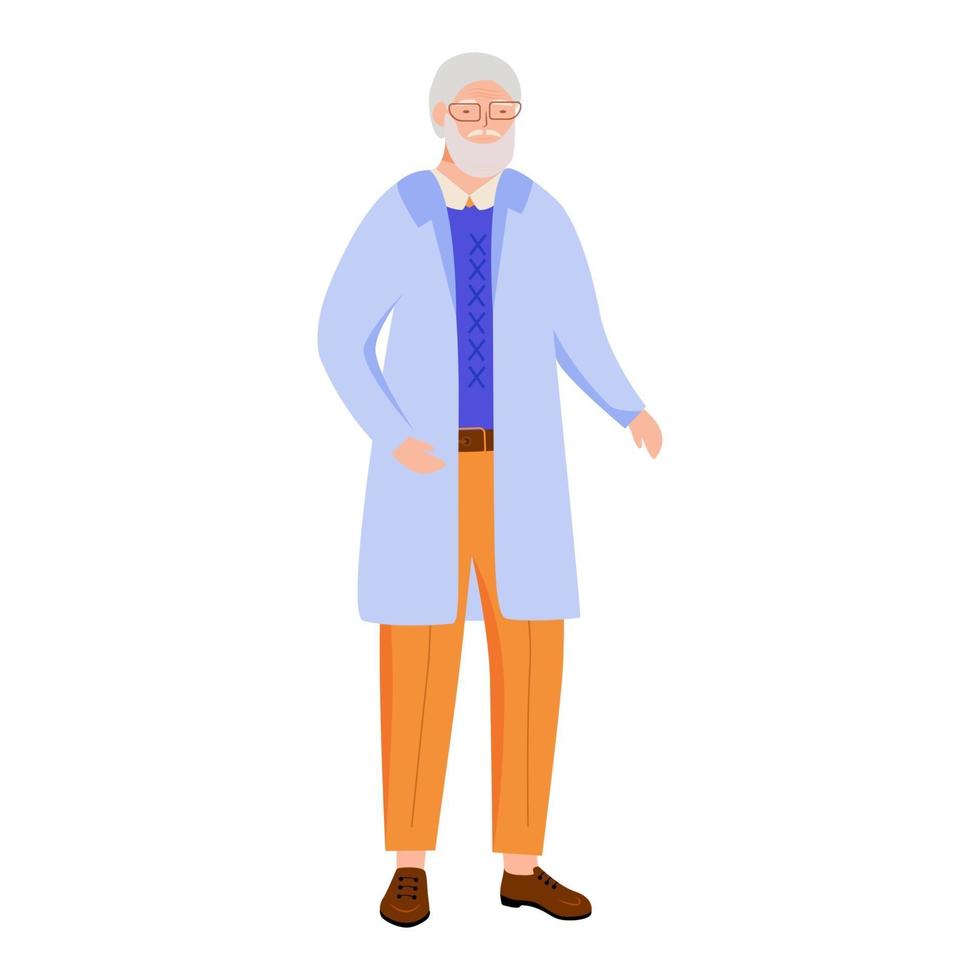The image is a digitally composed, cartoonish yet realistic illustration of an older man against a plain white background, giving the impression that the figure is floating. The man, who has short gray hair and a full beard extending into his chin, wears wire-rimmed glasses. His attire includes a light blue long coat that reaches halfway down his thighs, layered over a darker blue sweater, and under that, a white collared shirt with the collar peeking out. He is also sporting orange pleated pants that are slightly short, revealing his ankles, and a brown belt. His brown formal shoes have black laces. The man is facing forward but slightly turned to his left, with his arms at his sides in a raised position, suggesting either an impending gesture or the stiffness characteristic of old age.